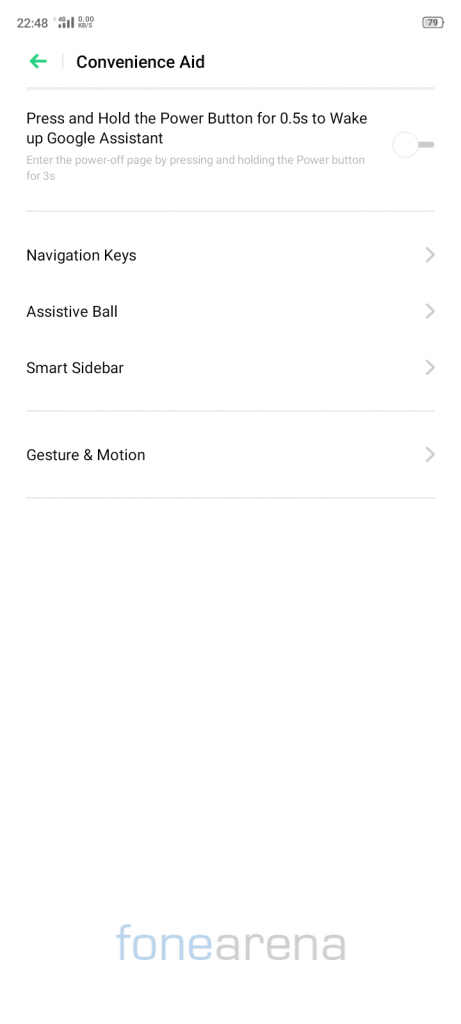This image is a screenshot taken on a mobile phone. In the upper left corner, the time is displayed in military format as 22:48, written in dark gray font. Adjacent to the time, signal strength bars are visible, indicating the phone's network reception. In the upper right corner, a battery icon, also in dark gray, shows a 79% charge with the percentage displayed inside the battery outline.

At the top center of the image, there is a bold black header that reads "Convenience Aid." To the left of this header, a green left-pointing arrow is present. Below "Convenience Aid," the text instructs, "Press and hold the power button for 0.5s to wake up Google Assistant," which is followed by a lighter gray text section.

Further down, additional menu options are listed including "Navigation Keys," "Assistive Ball," "Smart Sidebar," and "Gesture Motion." 

At the bottom of the screenshot, there is a potential watermark reading "fonearena." The word "fone" is written in a very light blue, while "arena" is in light gray. This text is enclosed in a rectangular box with a white background.